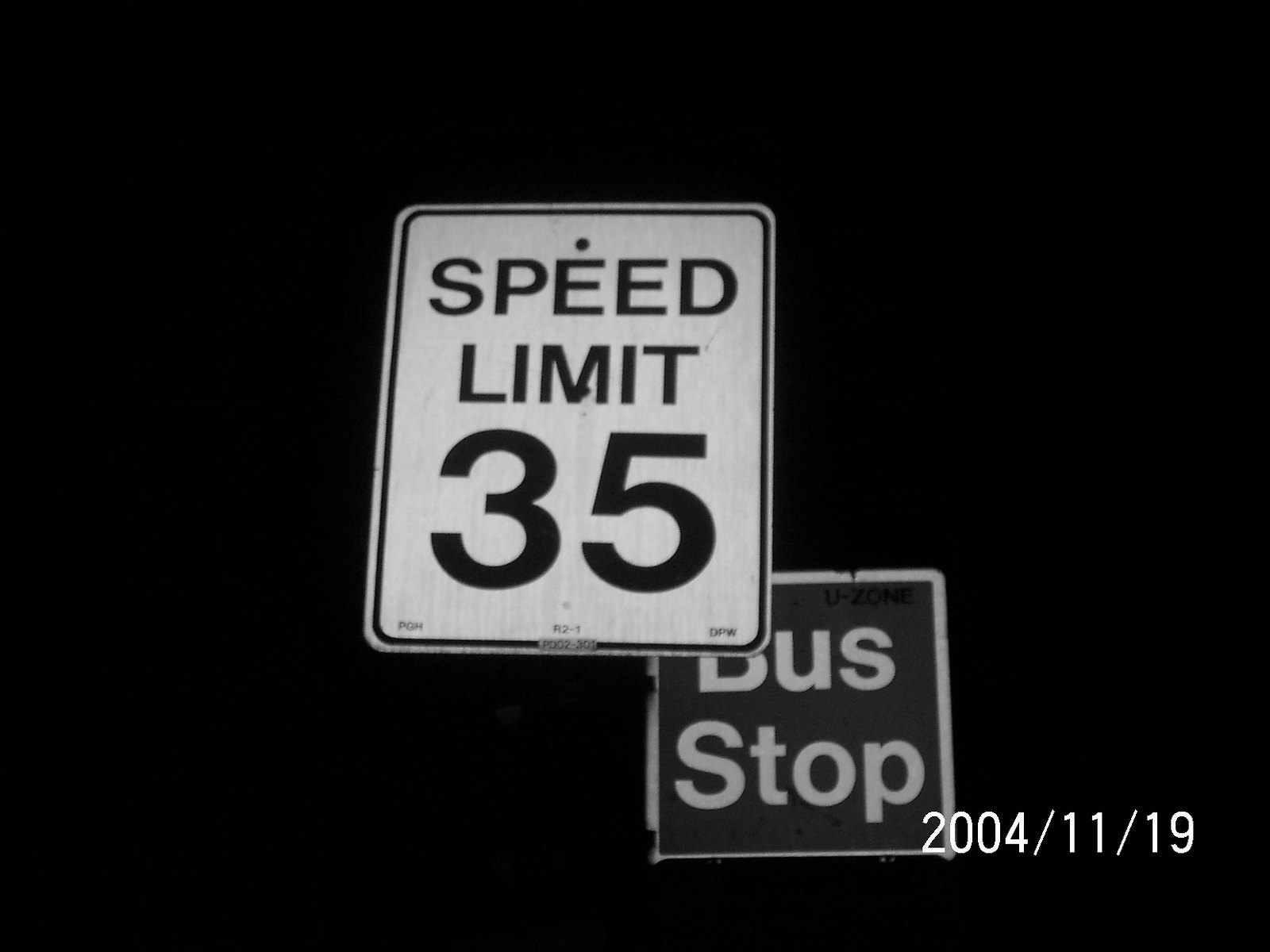Taken on November 19, 2004, this detailed image features a white speed limit sign indicating a maximum speed of 30 miles per hour. The sign, delineated with both a black and white trim, shows signs of weathering, including a hole above the first "E" used for attaching it to a pole and another hole in the middle of the letter "M." At the very bottom of the sign, there are small, unreadable words. Overlapping this speed limit sign is a bus stop sign in a grayish hue with white lettering, partially obscuring the letter "B." The 3D perspective of the photograph reveals not only the front but also the back of the signs, showing the structure and attachment mechanism, including a small box behind the bus stop sign.